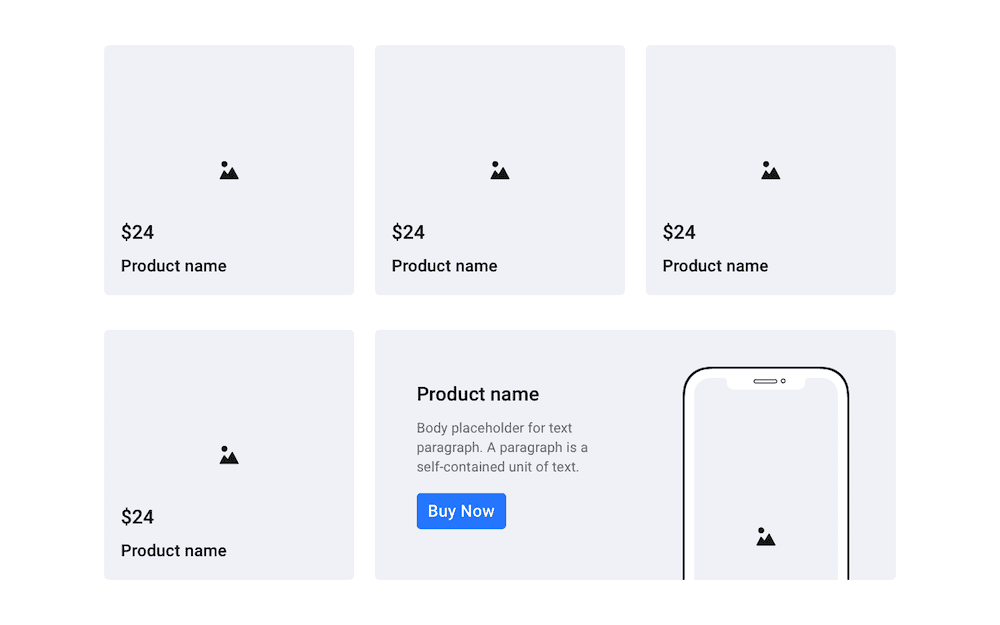In this image, we observe a layout consisting of five distinct tiles, each marked with a pin. The content of the tiles is as follows:
- The **first tile** displays the product name prominently.
- The **second tile** follows a similar format.
- The **third tile** continues this sequence.
- The **fourth tile** replicates the product name format.
- The **fifth tile** stands out, showing a mobile device with an empty thumbnail picture centered on its screen.

The color scheme of the image predominantly incorporates black, white, and blue tones. The fifth tile also contains placeholder text intended for a body paragraph, illustrating where additional information or a description would be placed.

In summary, this image highlights five key features or products with a uniform visual representation and a cohesive color palette, emphasizing the orderly presentation of information.